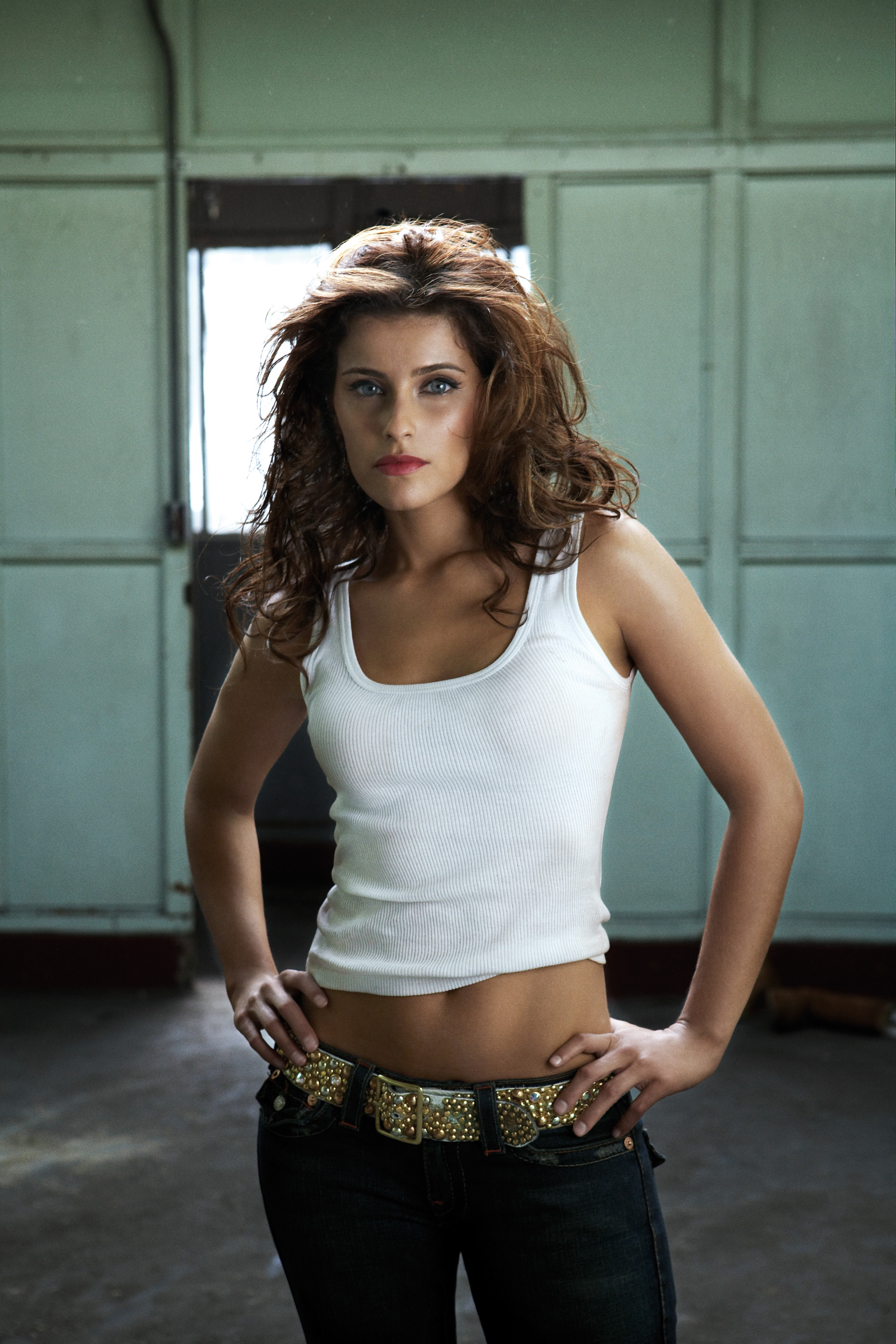In this image, a young white woman with long, dark curly hair is standing directly in the center, posing with her hands on her hips and looking straight at the camera with a stirring expression. She is wearing a white tank top that reveals part of her stomach, low-rise pants, and a shiny belt. Her makeup is heavy, emphasizing her features. The background consists of textured, wood-like square panels, likely part of a wall, with either a door or window just behind her head. The ground surface is a mix of gray and brown, suggesting it could be either hard flooring or carpeting. The setting appears to be indoors, possibly in a largely empty building, with a sense of daytime lighting. The overall color palette includes shades of gray, green, white, black, blue, gold, and silver, and there is no text present anywhere in the image.